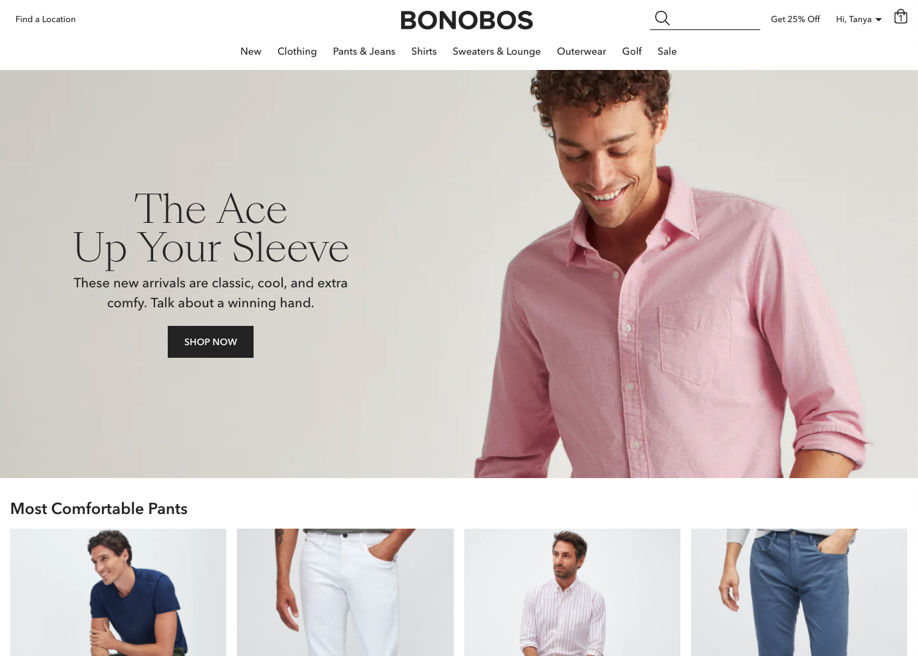This image depicts a retail webpage for Bonobos, a clothing line. At the top of the page, the Bonobos logo is prominently displayed in black and white. Below the logo, there is a navigational menu offering clickable options for categories such as New Arrivals, Pants & Jeans, Shirts, Sweaters & Lounge, Outerwear, Golf, and Sale items.

The main section of the page features a promotional image of a male model with short, curly brown hair, dressed in a pink shirt. Accompanying the image is the tagline, "The Ace Up Your Sleeve. These new arrivals are classic, cool, and extra comfy. Talk about a winning brand," along with a "Shop Now" button for immediate access to the featured products.

Further down, the webpage highlights "The Most Comfortable Pants" with a series of four images. The first image showcases a man wearing a blue t-shirt. The second image is a close-up of a white pair of pants. The third image features a different man wearing a striped dress shirt, while the final image is a close-up of some blue pants. These visuals illustrate various clothing options available from Bonobos, emphasizing comfort and style.